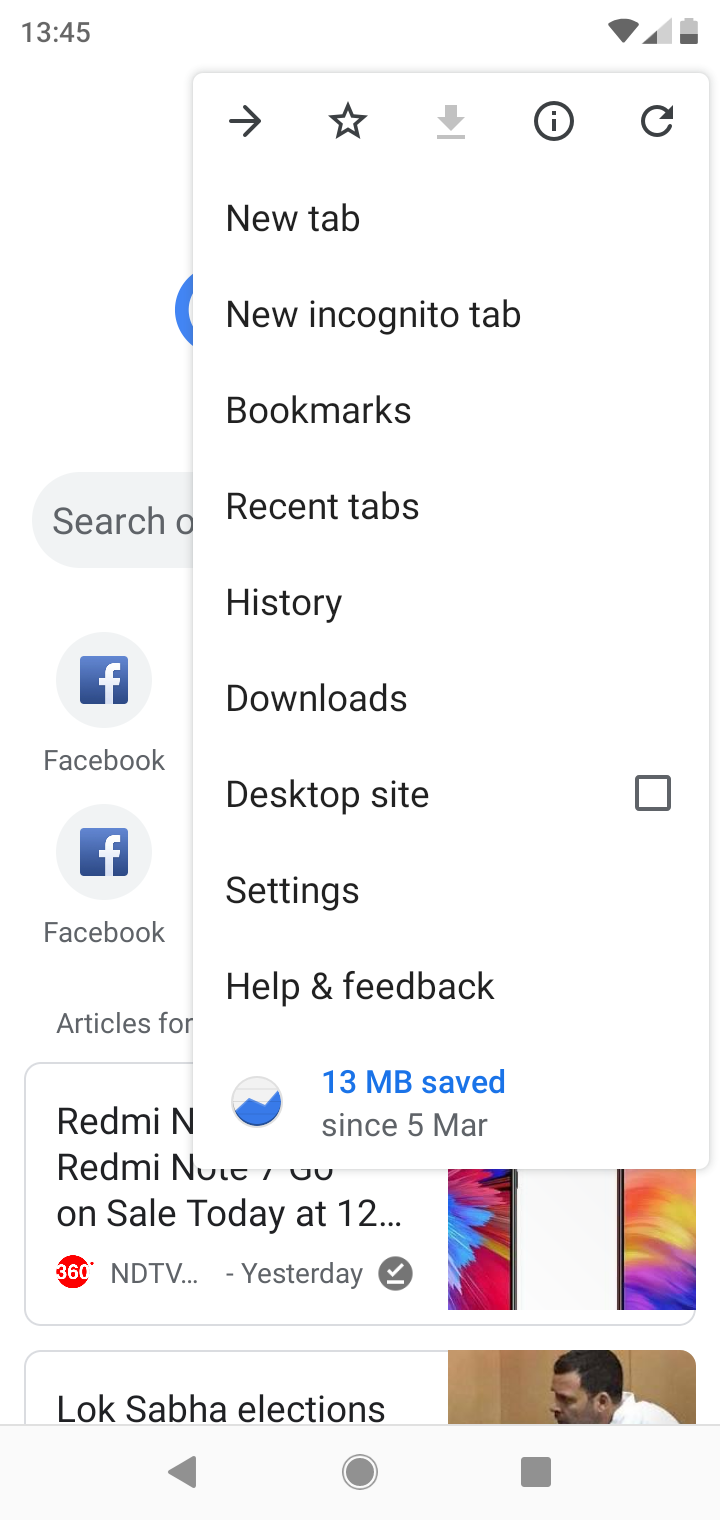The image displays a dialog box overlaid on a web browser interface. The dialog box, occupying the upper and lower sections, offers options such as "New tab," "New incognito tab," "Bookmarks," "Recent tabs," "History," "Downloads," "Desktop site," "Settings," and "Help & feedback." At the top of the dialog box, there are icons for navigation: a right arrow, a star, a download button (inactive), an eye with a circle, and a refresh symbol.

Behind the dialog box, the Google homepage is visible, showing the time "13:44" in the top left corner, and WiFi and battery icons in the top right corner against a white background. Below the dialog box, snippets of content can be discerned: a Google search prompt is visible, followed by thumbnails of frequently used apps, including two instances of Facebook. 

Beneath these, recent articles appear, with the first one from NDTV mentioning a sale, accompanied by a picture of smartphones. Another article is partially visible, displaying a person in a white shirt in court, mentioning the "Lok Sabha elections." The text is incomplete due to the overlaying dialog box. Additionally, a blue note indicates "13 MB saved since 5 of March."